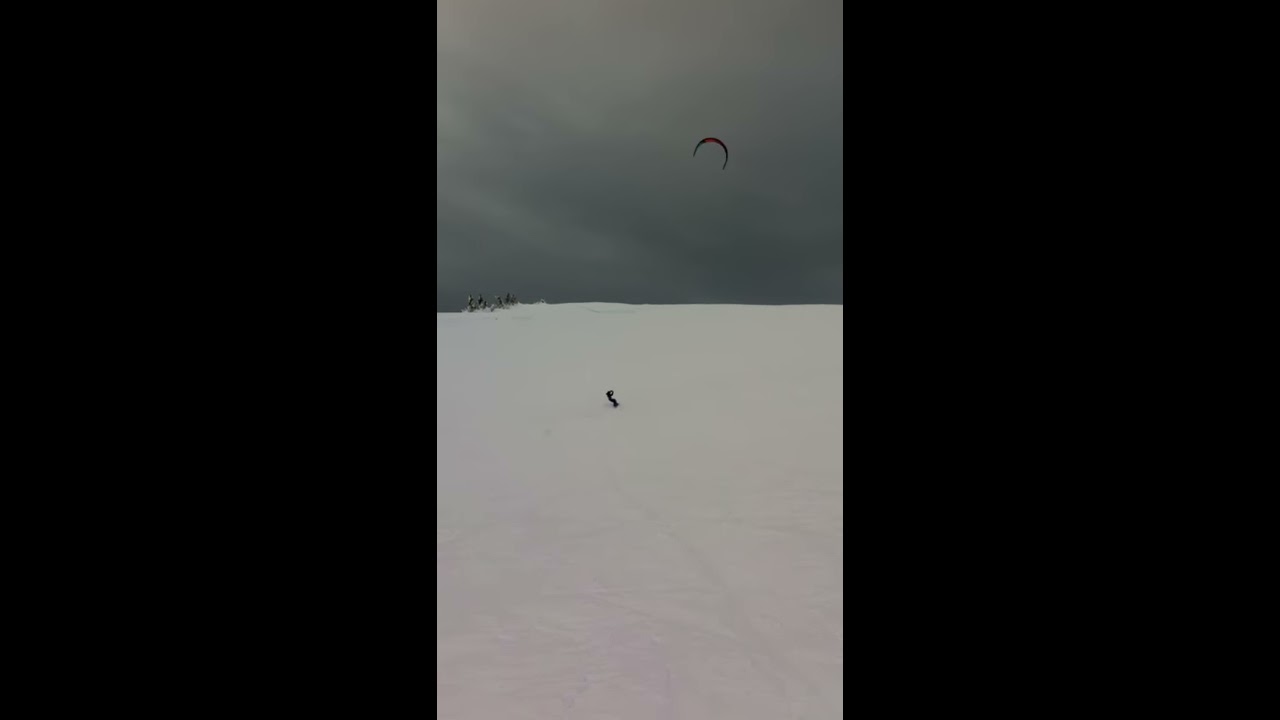The image depicts a winter scene captured outdoors under dark gray, overcast skies. The primary focus is on a snowboarder, albeit small and distant, who appears to be snowboarding down a steep, snow-covered hill using a parachute, suggesting an activity similar to wind snowboarding or snow kiting. The largely white and wintry landscape contrasts with the gloomy, cloud-covered sky. Far off in the distance to the left, faint rocky mountains are partially visible, adding depth to the overcast and somber atmosphere. The composition of the photo is vertical, which emphasizes the height of the hill and the expansive, dark sky overhead.